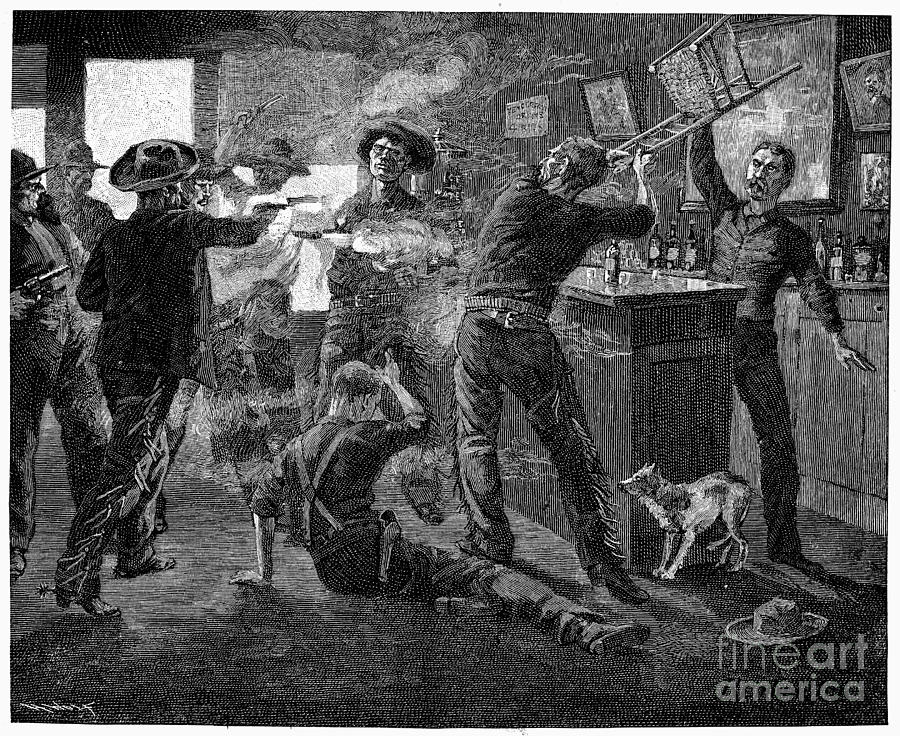This detailed black and white drawing, likely created with charcoal or pen and ink, vividly depicts a chaotic bar fight in an Old West saloon. The scene is rich in action and detail, capturing a moment of intense brawling involving seven men. To the right is a wooden bar top, adorned with pitchers and bottles of alcohol, set against a backdrop of a large mirror and several hanging portraits. The bartender, distinguished by his vest and pants, and sporting a large handlebar mustache, is reaching up to grab a chair, trying to prevent a man from swinging it at another individual across the bar. At the bartender's feet, a frightened small dog cowers with its tail between its legs, adding a touch of vulnerability to the chaotic scene.

Nearby, a cowboy hat lies abandoned on the floor, and the watermark "Fine Art America" is notably present in the bottom right corner, with 'Fine' in thinner print than 'Art America'. Multiple men off to the left are depicted firing their guns, with smoke wafting across the image, contributing to the sense of pandemonium. One man stands with his back to the bar, appearing to have just been shot, while another man lies on the ground in front, possibly having been knocked down during the fray, with a hand on his head and wearing a dark shirt with white suspenders. The detailed shading and dramatic composition bring the tumultuous energy of an Old West bar fight to life.